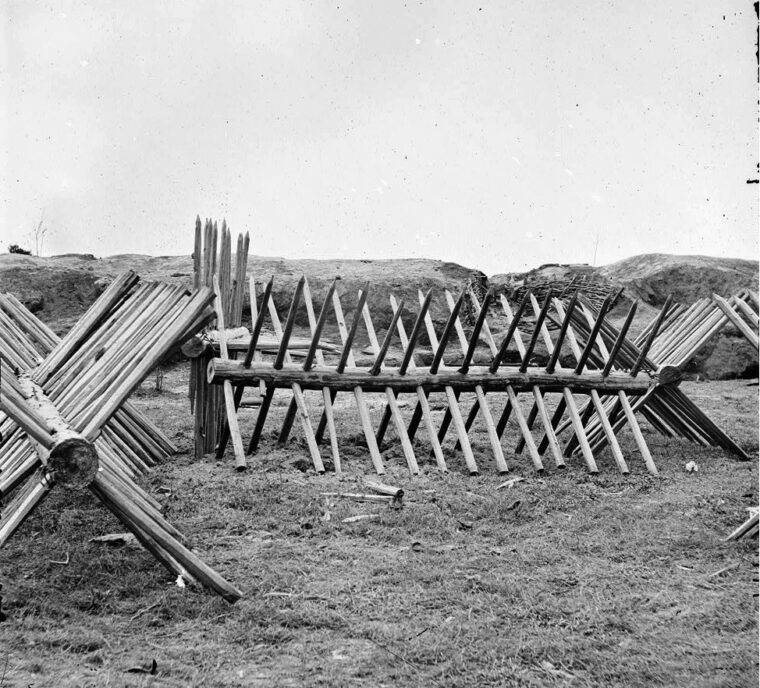This black and white square photograph captures a grassy field under an overcast sky, possibly stormy. The central focus is on several wooden barricades, arranged in X-shaped formations created by perpendicular stakes protruding from large horizontal logs. These structures, likely resembling pike barriers from war times, are aligned in rows—one long rack on the left, one central, and another partially visible on the right. The foreground shows two to three prominent barricades, with additional ones discernable in the distance, partially obscured. Some of the stakes appear to be sharpened to points, giving a menacing look to the scene reminiscent of Civil War reenactments. The background features dirt banks and rocky hills, adding depth to this grainy, vintage photograph.